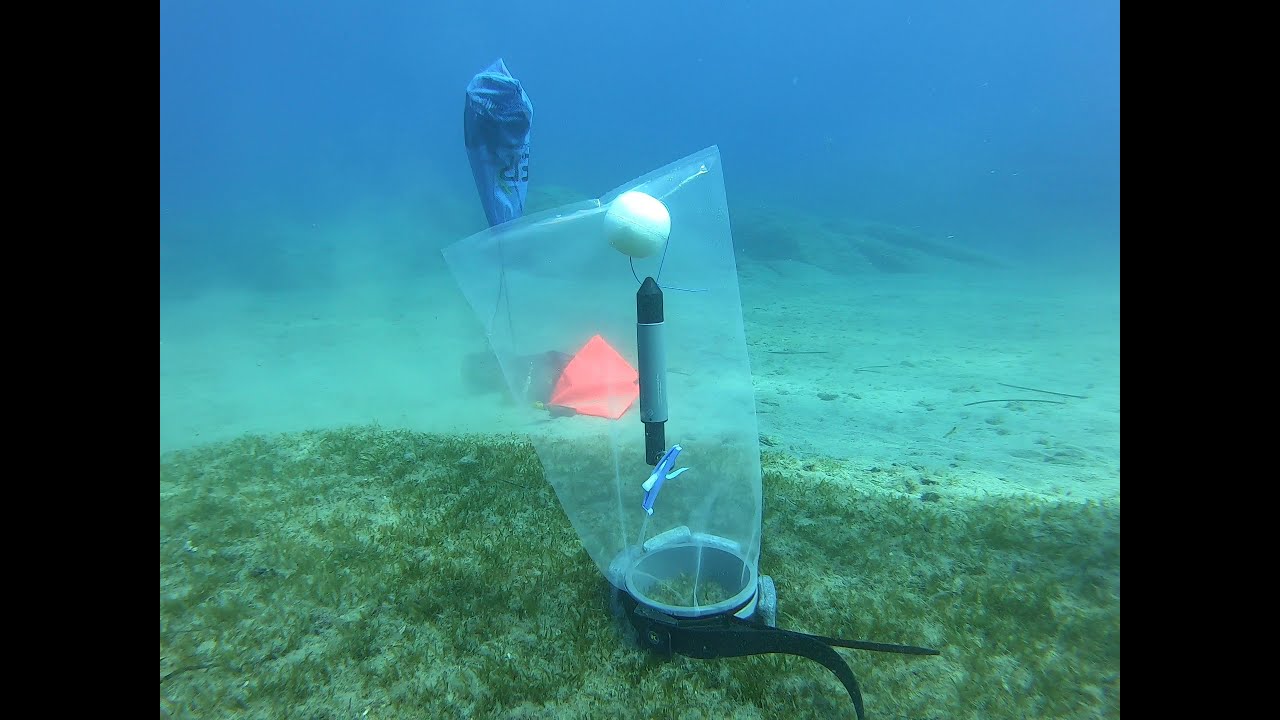This underwater photo has a horizontally aligned rectangular shape with thick black vertical borders, making the central colored image appear more square. It reveals a serene, blue-tinted ocean floor characterized by a flat, sandy terrain interspersed with occasional bumps and small grain-like plants in the foreground. Central to this image is a curious arrangement of objects within a plastic bag. Inside the bag, a white round object floats upwards, tied to a narrow black and gray cylinder, which in turn is connected to a blue cylinder object. The base of this assemblage is anchored by a gray and black wristband, held in place by several rocks. Nearby, a blue duffel bag appears to be floating upwards as well, tethered to two square black objects. The background showcases more of the sandy ocean floor, adding to the mystique of this seemingly scientific setup, potentially meant for recording or study, amidst what appears to be seaweed and oceanic sand.